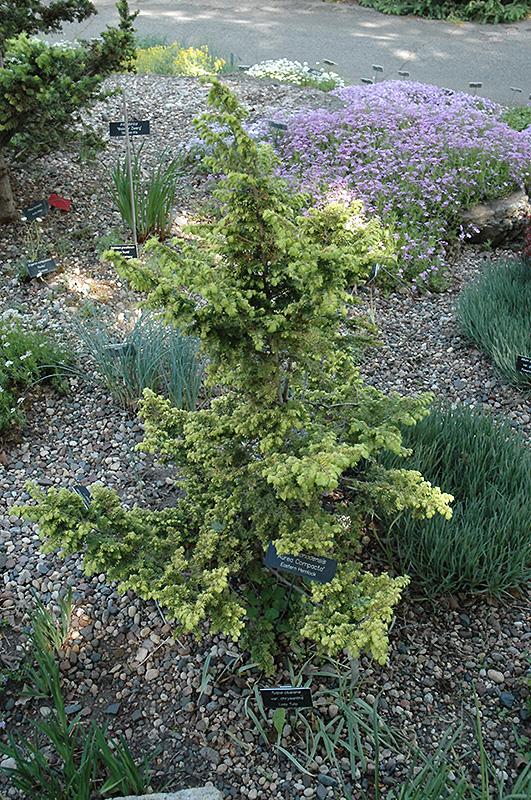The image displays a serene outdoor scene, likely within a botanical garden or park area, showcasing a variety of meticulously labeled plants and trees. Central to the image is a small, green tree identified as Aurea compacta or Eastern Hemlock, accentuated by its robust, green shoots. Surrounding this focal tree, there are patches of diverse vegetation, including purple and pink flowers, as well as various grasses that contribute to the garden's rich tapestry of colors—black, gray, green, purple, pink, and red. The soil around the plants is covered with small, rounded gray and white pebbles, adding texture to the scene. In the background, additional trees and vibrant flora can be seen, along with an asphalt-paved walking path bordered by white flowers, inviting nature enthusiasts to explore further. The image is bathed in daylight, suggesting a bright, sunny day, enhancing the vividness of the greenery and the overall tranquility of this garden setting.